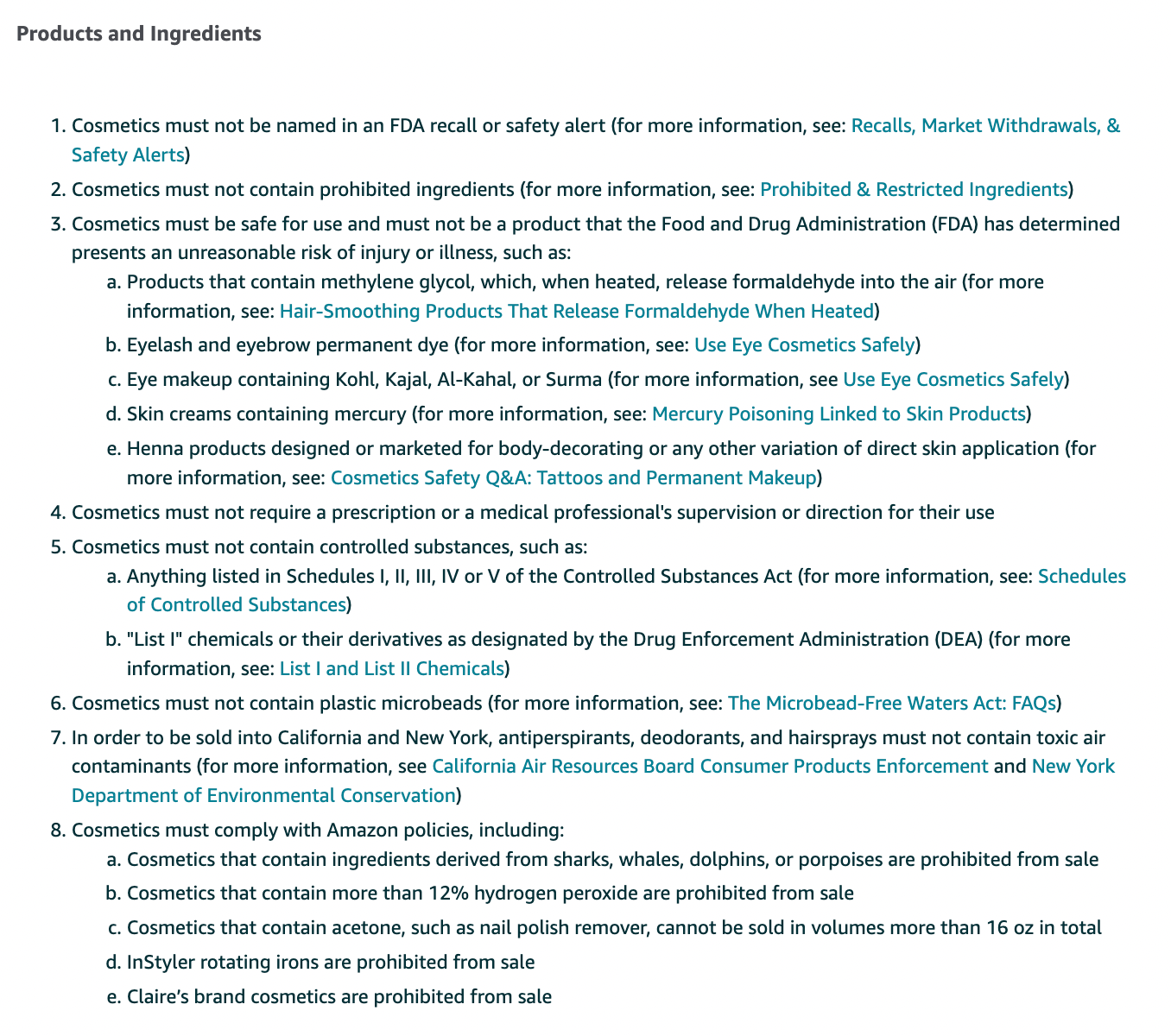The image contains a detailed passage of information regarding cosmetics and their ingredients, displayed on a white background with black text. Highlighted sections, where clickable links are available, are shown in blue. The passage covers several critical aspects of cosmetic safety regulations, outlined as follows:

1. **FDA Recalls and Safety Alerts:** Cosmetics must not be named in an FDA recall or safety alert. For additional details, refer to the section on recalls, market withdrawals, and safety alerts.
2. **Prohibited Ingredients:** Cosmetics must not contain any prohibited ingredients. Further information can be found in the section on prohibited and restricted ingredients.
3. **Product Safety:** Cosmetics must be safe for use and must not present an unreasonable risk of injury or illness, such as products containing methylene glycol, which releases formaldehyde when heated. More information is available in the section on hair smoothing products that release formaldehyde when heated.
4. **Eyelash and Eyebrow Dyes:** Specific information on permanent dyes for eyelashes and eyebrows can be found under the section on using eye cosmetics safely.
5. **Eye Makeup Ingredients:** Products containing kohl, kajal, alcohol, or serma should also be used safely. Additional details are provided in the use eye cosmetics safely section.
6. **Mercury in Skin Creams:** Skin creams containing mercury are addressed, with further information available in the mercury poison linked to skin products section.
7. **Henna Products:** Henna products marketed for body decoration or any direct skin application are discussed, with more information available in the cosmetics safety Q&A, tattoos and permanent makeup section.
8. **Prescription and Controlled Substances:** Cosmetics should not require a prescription or medical professional's supervision and must not contain controlled substances listed in Schedules 1, 2, 3, 4, or 5 of the Controlled Substances Act. More details can be found in the schedules of controlled substances section.

This comprehensive guide ensures consumers are well-informed about the safety requirements and prohibited substances in cosmetic products.